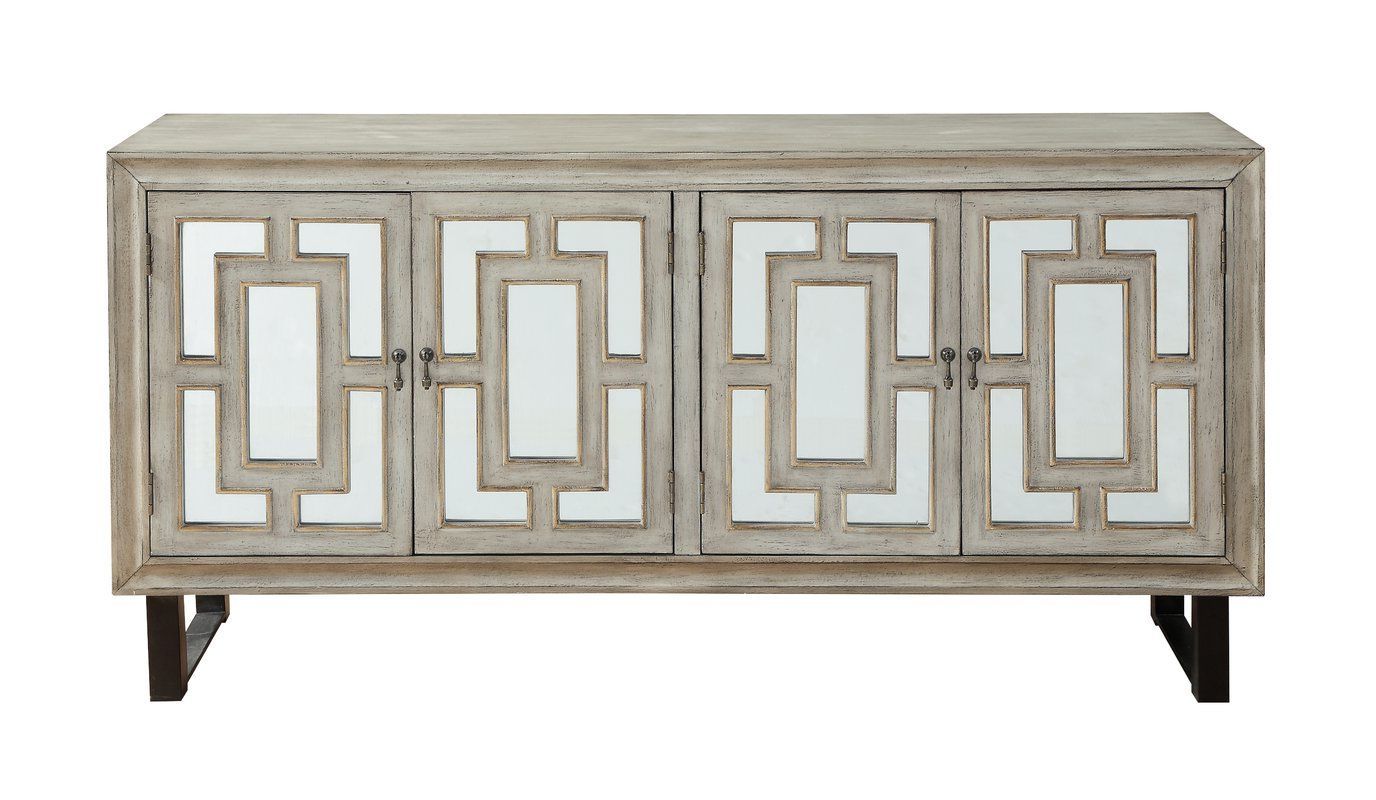The image is a color photograph featuring a credenza against a plain white background. The credenza is made from a light beige picklewood, showcasing a wood grain pattern. It has a rectangular shape and stands on black, square-tube legs. The front of the credenza is outfitted with four doors, each featuring black knobs for opening. The doors have a chic design: a white inset rectangle is framed by the picklewood, with an elegant L-shaped border at both the top and bottom. Additionally, each door has visible black hinges, adding to its detailed craftsmanship. Overall, the piece exudes a rustic yet modern aesthetic, making it a versatile addition to any room.